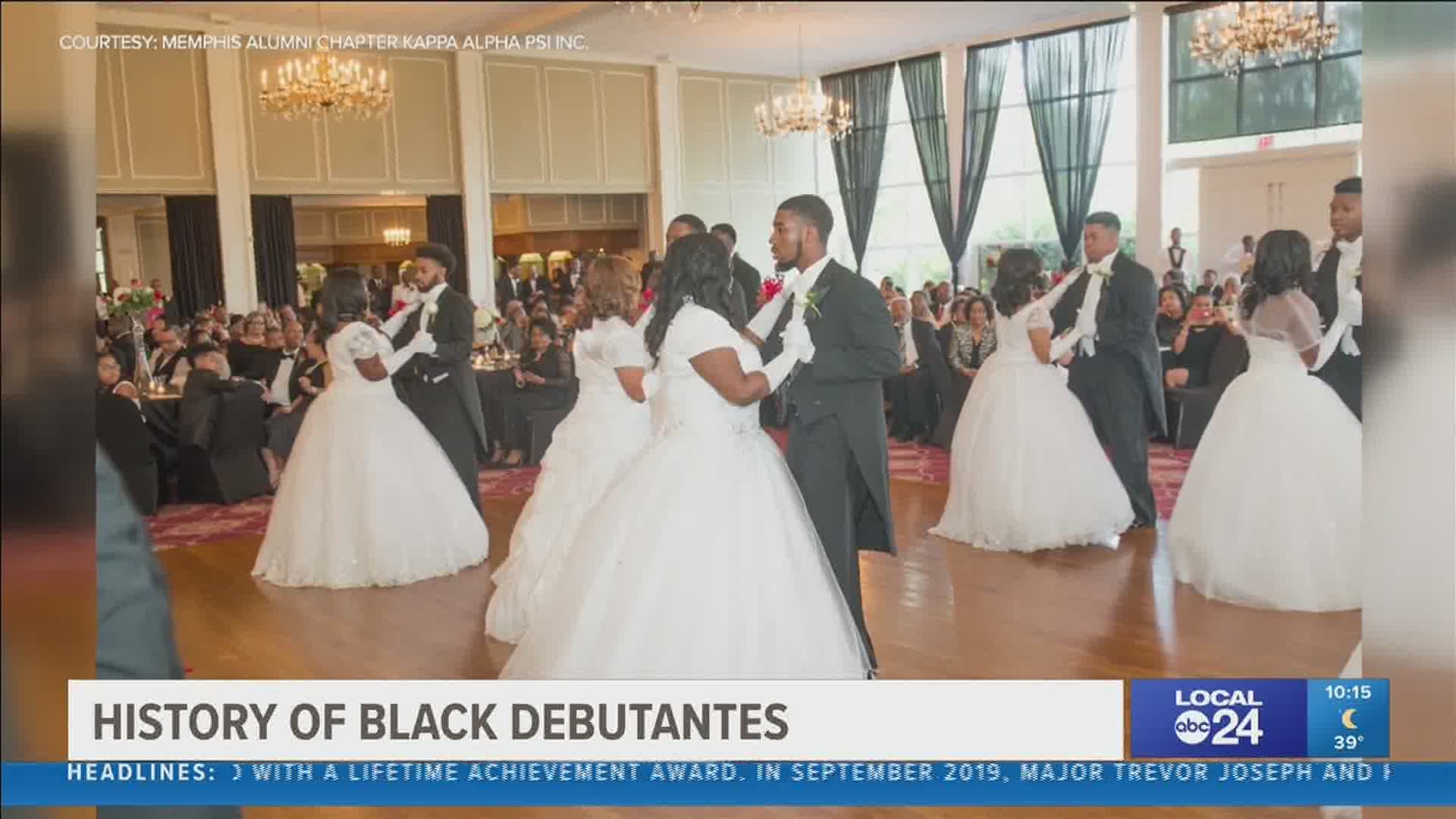This image is a detailed capture of a news report, showcasing an elegant dance event. At the upper left of the screen, white text reads, "Courtesy Memphis Alumni Chapter Kappa Alpha Psi Inc." On the bottom left, black text on a white rectangle states, "History of Black Debutantes." A chyron beneath it indicates, "Headlines with a Lifetime Achievement Award in September 2019 Major Trevor Joseph and I," though part of the message is cut off. On the right, within a blue rectangle, it says "Local ABC 24," and below that in a lighter blue square, "10:15," next to a crescent moon and the temperature of 39 degrees. 

The actual photograph at the center of the screen portrays a group of African-American men and women dancing in a sophisticated ballroom. The men are dressed in black tuxedos, while the women wear elegant white gowns and gloves, with their hair down. The ballroom is adorned with chandeliers and large green curtains covering the windows. Seated at tables around the dance floor, a large audience watches the dancers, adding to the grandeur of the event.